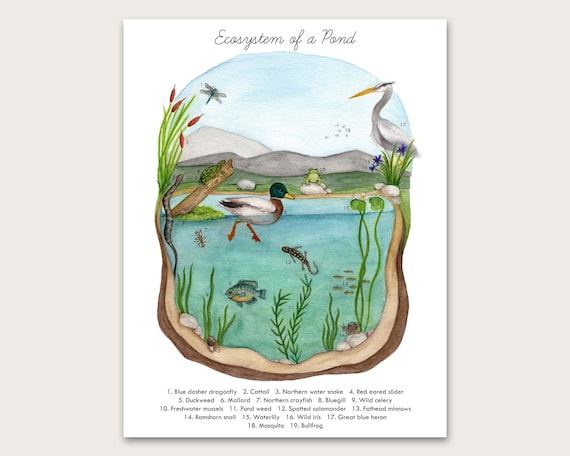The image portrays a page that appears to be from a book or educational resource, set on a gray rectangular background with a white vertical rectangle in the center. At the top of the white page, the title "Ecosystem of a Pond" is elegantly scripted in cursive writing. Dominating the white space is a vibrant, watercolor-style, artistic depiction of a diverse pond ecosystem, bursting with colorful, rounded imagery.

In the pond scene, central attention is drawn to a duck swimming gracefully through the transparent water. Around it, a myriad of pond life is teeming: a turtle scales a piece of wood, a snake emerges from the water, and a fish swims below the duck, with plants such as cattails and seaweed rising from the pond's depths. To the right, a large white bird, possibly a heron, stands majestically. Dragonflies flit near the surface while a frog perches on a stone, encapsulating the rich biodiversity of the pond.

Beneath the illustrated scene is a detailed numbered list identifying the various flora and fauna depicted. This includes:

1. Blue dasher dragonfly
2. Cattail
3. Northern water snake
4. Red-eared slider
5. Duckweed
6. Mallard
7. Northern crayfish
8. Bluegill
9. Wild celery
10. Freshwater mussels
11. Pondweed
12. Spotted salamander
13. Fathead minnows
14. Ram's horn snail
15. Water lily
16. Wild iris
17. Great blue heron
18. Mosquito
19. Bullfrog

The chaotic yet harmonious mix within the pond scene brings to life the interconnectedness of these species and their habitat, making this page a vivid tribute to the intricate ecosystem of a pond.